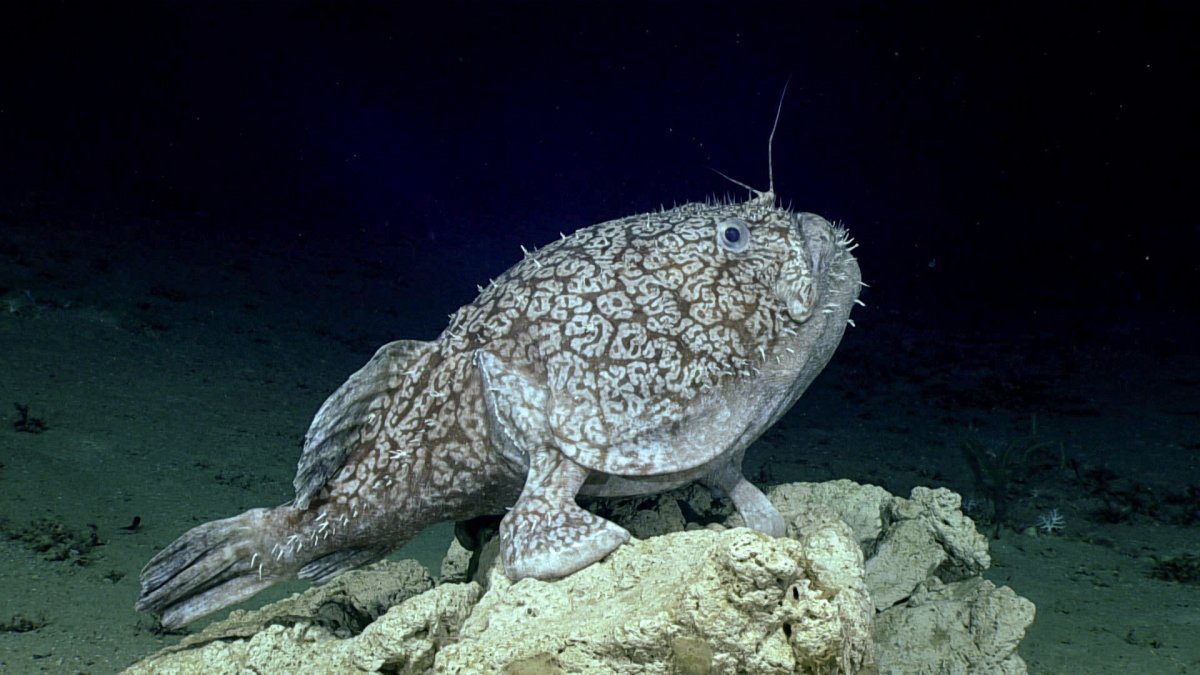The image captures an underwater scene with a clear view of a distinctive sea creature positioned centrally. This creature, likely a fish, features an oval-ish, rounded body with a tapering tail fin. The fish is standing on white rocks or coral at the sandy bottom of a body of water. The background displays a dark blue, giving an impression of depth, while the foreground includes sparse green plants, similar to seaweed, scattered around.

This fish has a brown body adorned with a white design resembling coral, aiding in its camouflage. A prominent tail fin touches the sandy floor, and just to the right of this fin is a smaller gray and white fin. Interestingly, it possesses small antennae projecting from its head near its round white eye with a black center. Below the mouth, there are small, white-like protrusions that resemble hairs, set against a light gray underbelly. The scene around the fish is serene, hinting at a natural underwater habitat possibly photographed by a wildlife photographer.